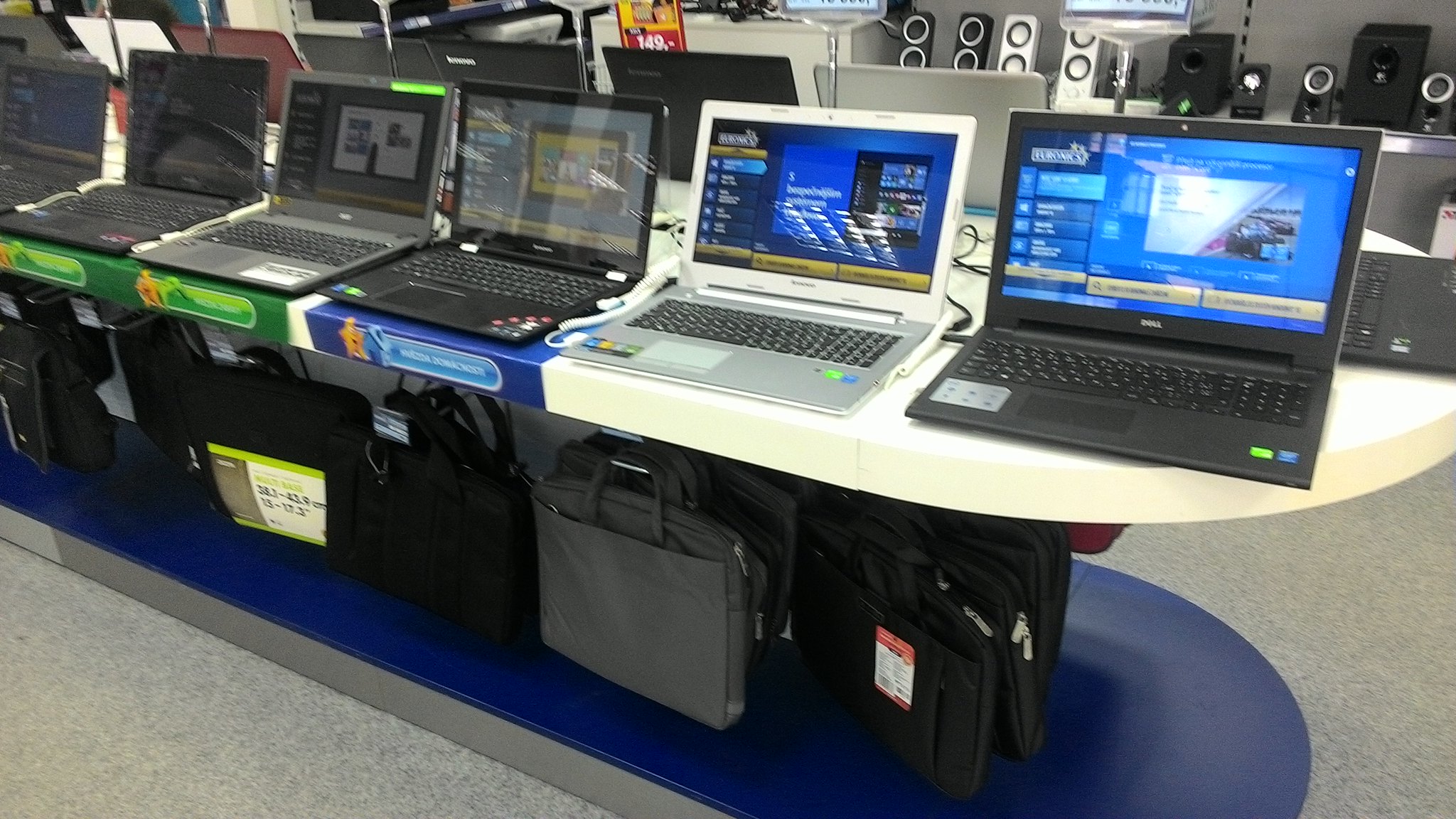The image depicts an interior view of an electronic store, featuring a white counter with a blue base that is rounded at the right end. Atop the counter, a variety of open laptops are neatly positioned in rows. The laptops come in different colors, including black, white, gray, and silver, each displaying different images on their screens. In front of a few laptops, labels are visible, and there is a red and yellow sales tag on one of them. The counter sits on a gray stone floor, with several laptop bags or backpacks stored underneath, each dedicated to a corresponding laptop. In the background, various speakers of different sizes and colors, predominantly black and one white, are displayed on another counter. This detailed setup suggests that the photo was taken in a retail store, likely a well-known electronics store, such as Mediamarkt.